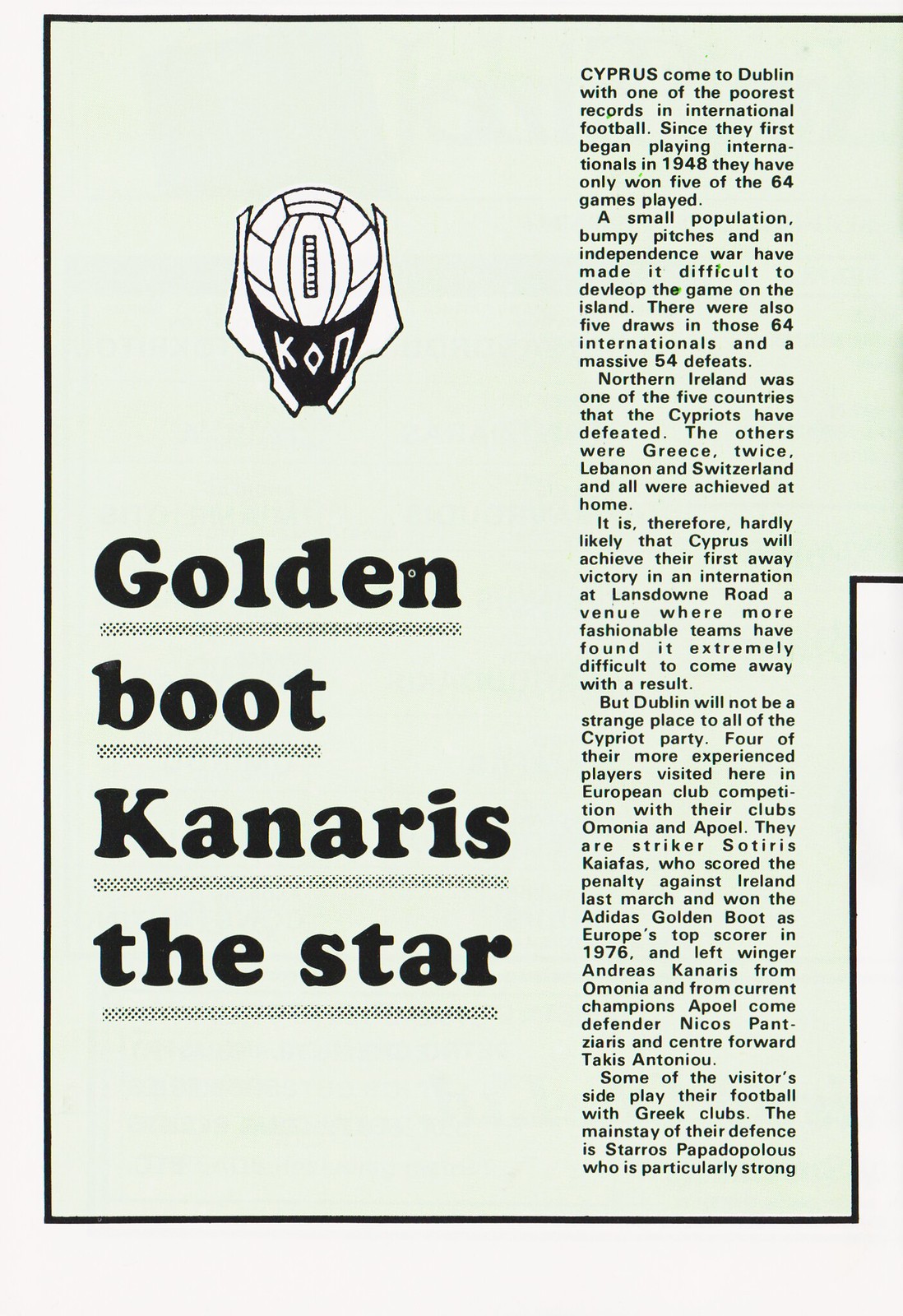The image features a magazine-style page set against a tan and white background. At the top, there's a stylized geometrical logo with "KON" inscribed in it. Below the logo, large bold black letters proclaim the headline: "Golden Boot Canaris the Star." The article that follows is formatted in a single, right-justified column of smaller print on the left side of the page. The text details the struggles and achievements of Cyprus in international football since their first games in 1948, highlighting their record of only five wins out of 64 games, with five draws and 54 defeats. Factors such as a small population, bumpy pitches, and an independence war have hindered football development on the island. Notable victories included Northern Ireland, Greece (twice), Lebanon, and Switzerland. The article also mentions that Cyprus is unlikely to secure their first away victory at Dublin's Lansdowne Road, a challenging venue even for more established teams. However, some of the Cypriot players are familiar with Dublin from European club competitions, including striker Sotiris Caiaphas, who won the Adidas Golden Boot in 1976 as Europe's top scorer, left winger Andreas Canaris, defender Nikos Pantisarias, and centre-forward Takis Antoniou. Staros Papadopoulos, a strong defender, is also highlighted. The page features a mix of colors including white, tan, black, light green, and gray.